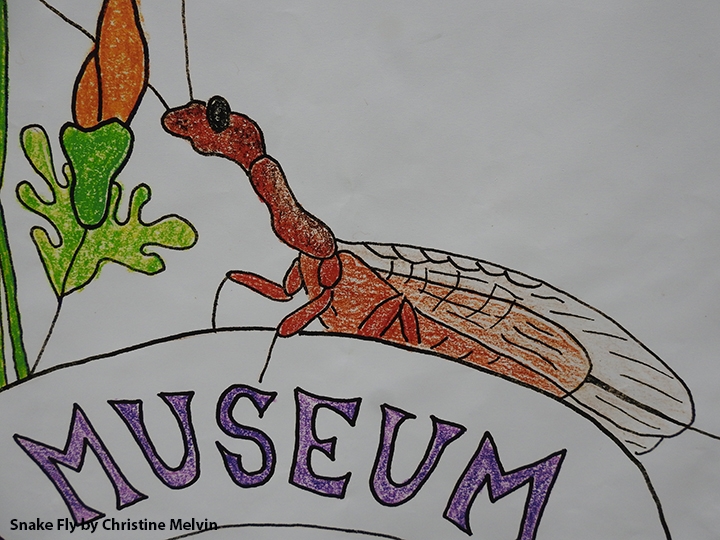The image is a detailed photograph of a crayon-colored drawing titled "Snakefly by Christine Melvin," as indicated by the text at the bottom left. The central focus is a brownish-red insect, resembling a snakefly, characterized by a head with antennae, a long neck, legs, a rather elongated body, a tail at the end, and large, transparent wings. The insect is positioned in the middle, with its head pointed towards the top left. It stands on a white arch that has the word "Museum" inscribed in purple text. Adjacent to the insect, on the right, is a plant with green leaves and an orange bud, likely representing some kind of vegetable. The background is predominantly gray, with portions blending into white. The drawing encapsulates a kid's coloring book aesthetic, with the use of vivid colors such as yellow, green, darker green, orange, brownish-red, purple, white, black, and gray.